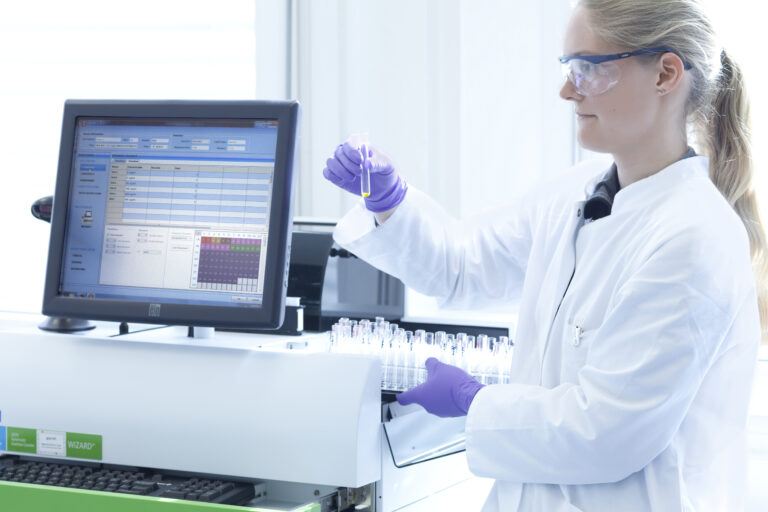The image captures a bright and clear laboratory scene, featuring a woman with a light complexion and long blonde hair tied back in a ponytail. She is dressed in a white lab coat, blue-framed protective goggles, and purple latex gloves. The woman stands on the right side of the picture, holding up a test tube containing a small amount of yellow liquid in her right hand, and a tray filled with more test tubes in her left hand. To her left, on a table, there is a rectangular computer screen displaying a table or chart, although the specific content is illegible. Below the screen, there is a keyboard, and the frame of the monitor has green stickers, including one that reads "wizard." The laboratory background features white walls and windows, bathed in natural light, contributing to the image's overall clarity.